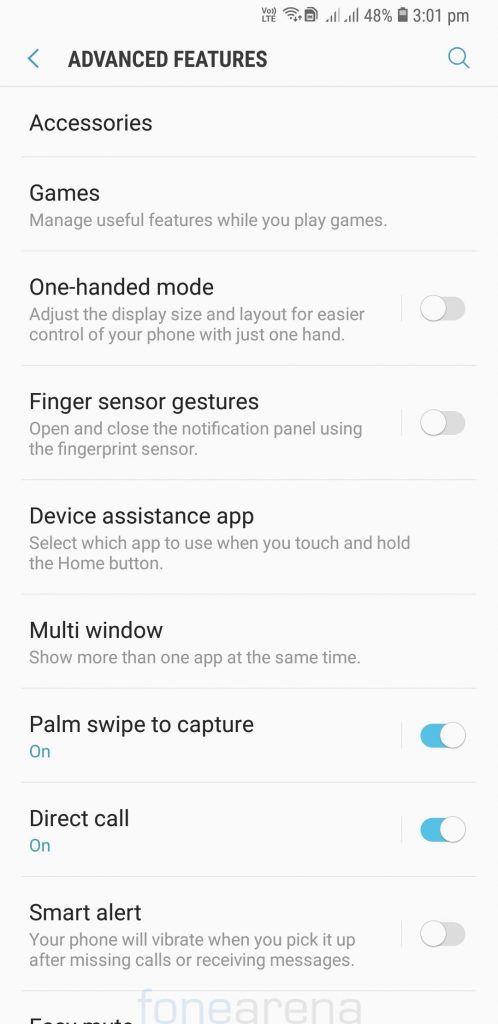**Screenshot of Advanced Features Settings on a Smartphone**

This screenshot captures the advanced features settings of a smartphone, displayed on a white background. At the top right corner, a status bar shows an array of system indicators including the time, battery percentage, Wi-Fi signal strength, data signal, and an LTE icon.

Dominating the top left of the screen, in bold black letters, is the title "Advanced features," accompanied by a blue left-pointing arrow and a magnifying glass icon to the right. Below this header, the settings are organized under various categories:

1. **Accessories** 
2. **Games:** Beneath this, a brief description reads, "Manage useful features while you play games."
3. **One-handed mode:** In black text, this is followed by a gray description, "Adjust the display size and layout for easier control of your phone with just one hand." A toggle switch to the right of this feature shows that it is currently turned off.
4. **Finger sensor gestures:** A description is provided below it, along with a toggle switch positioned on the right, which is also turned off.
5. **Device assistance app**
6. **Multi-window**
7. **Palm swipe to capture:** The toggle for this feature is turned on.
8. **Direct call:** Another feature with its toggle switched on.
9. **Smart alert:** This is listed at the bottom of the screen.

The overall layout is user-friendly, providing concise descriptions for each feature and visual indicators for their current activation status.